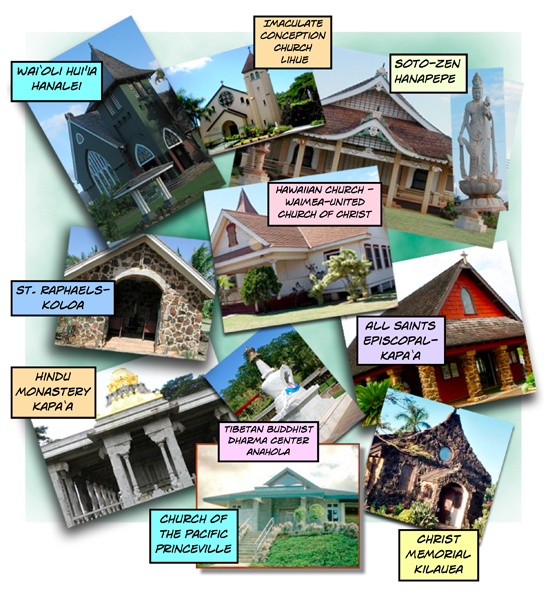The image is a digitally created collage featuring photographs of various buildings in Hawaii. Each building's name is displayed on a colored rectangle with black print. The collage, set against a light green background, is approximately four inches wide and four to five inches tall. At the 12 o'clock position, a church labeled "Immaculate Conception Church Lihue" in black print on a light orange square is shown. Moving clockwise, "Soto Zen Hanapepe" is on a cream rectangle, followed by "Hawaiian Church Waimea - United Church of Christ" on a pink rectangle. "All Saints Episcopal Kapa'a" is shown on a blue rectangle, and "Christ Memorial Kilauea" is below it. At the six o'clock position, "Church of the Pacific Princeville" is presented on a light blue rectangle, with "Tibetan Buddhist Dharma Center Anahola" directly above it. Positioning continues with "Hindu Monastery Kapa’a" on a light tan rectangle at the eight o'clock position and "St. Raphael's Koloa" on a stone house at the nine o'clock position. Finally, at the 11 o'clock position, there is another church’s name, "Waioli Hui-Aia Hanalei", on a rectangle. The collage features a mix of blue skies, stone, brown, white, green, light blue, gray, yellow, and red colors, indicating that the photos were taken outdoors during the daytime. The text is in black print and varies by language and color.